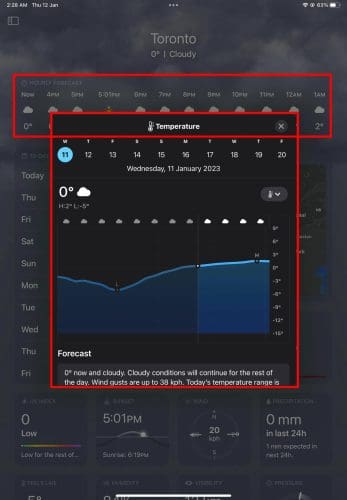The image features a gray background with weather information for Toronto, displaying a temperature of zero degrees Celsius and cloudy skies. The day is Thursday (THU), the 12th of January (JAN). A red rectangle highlights key times from 4 p.m. to 1 a.m., which includes specific marked hours: 4 p.m., 5 p.m., 6 p.m., 7 p.m., 8 p.m., 9 p.m., 10 p.m., 11 p.m., 12 a.m., and 1 a.m. At 5:30 p.m., there is a symbol of the sun breaking the cloud sequence.

Under "Now," the temperature is listed as zero degrees and rises to two degrees by 1 a.m. The rest of the temperatures for the highlighted hours are obscured by a pop-up box. The pop-up box displays numbers from 11 to 20, and the days abbreviated by their initials "M" for Monday, and the rest of the week's initials: "T" (Tuesday), "W" (Wednesday), "T" (Thursday), "F" (Friday), "S" (Saturday), with symbols indicating the weather. The 11th has a blue circle behind it, representing a highlighted date, and the sequence of days repeats across the display.